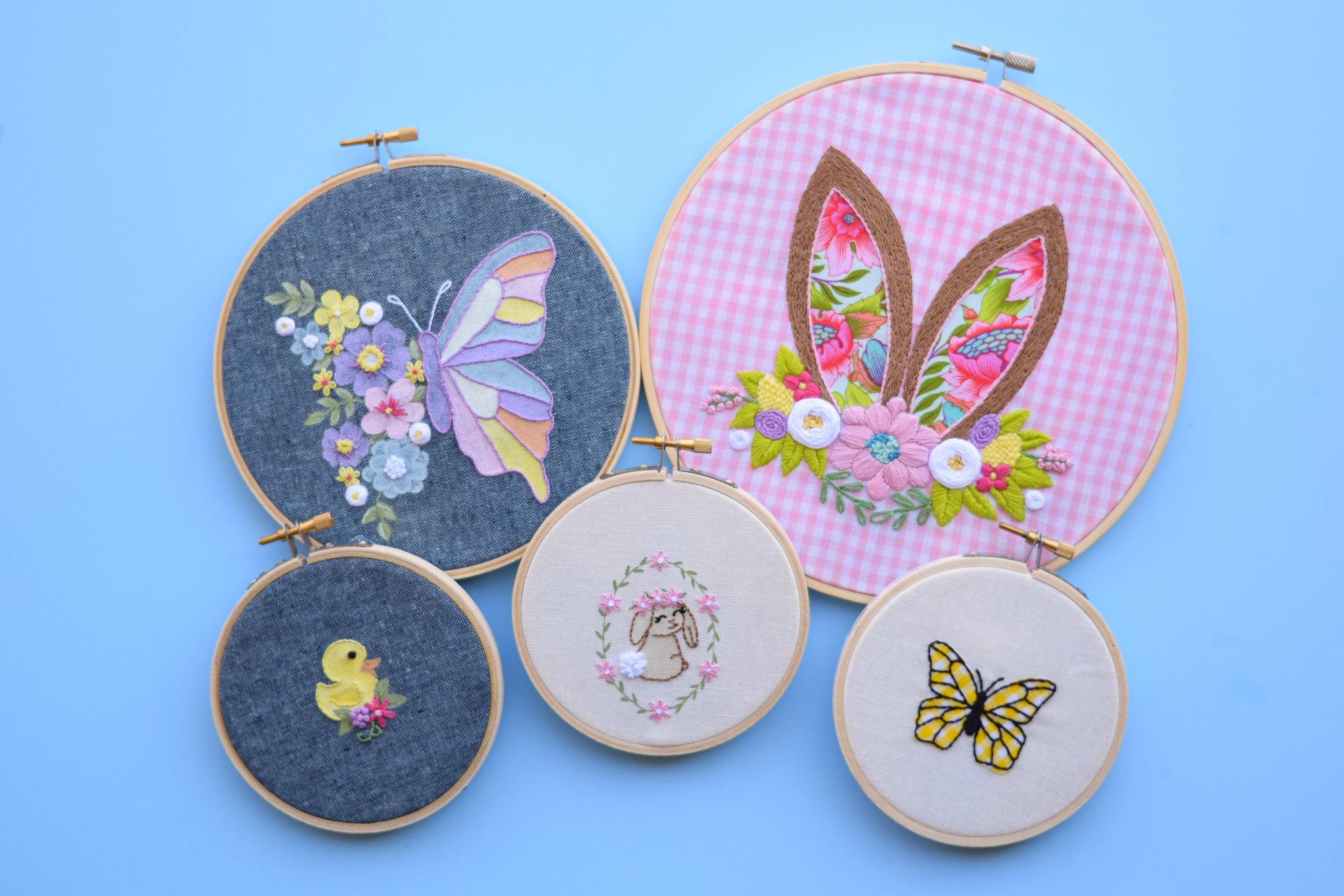This landscape-oriented color photograph showcases five meticulously crafted embroidery hoops, each featuring a unique, hand-stitched design evocative of a quaint and cozy aesthetic. All the designs are housed inside wooden hoops arranged against a light blue background. In the top row, on the left, there is a large hoop with a butterfly pattern, its wings composed of multicolored segments, set against a denim blue fabric and adorned with button trims and floral appliqués. On the top right, another large hoop displays a pair of bunny ears, stitched onto a pink and white gingham background, accented with floral patterns inside the ears and button trims underneath, accompanied by embroidered flowers. 

Below, three smaller hoops present animal-themed designs central to the image: on the bottom left, a cheerful yellow duckling stitched onto a blue fabric; in the center, a cream-colored baby rabbit meticulously crafted on a white background; and on the bottom right, a vibrant yellow butterfly occupying the hoop, also set against a blue background. The craftsmanship and detailed needlework, which include elements of appliqué and various materials, demonstrate a blend of realism and artistic representation. This warm and inviting collection predominantly features motifs suggestive of Easter themes, with each hoop individually adjustable by a screw at the top, emphasizing their functional as well as aesthetic qualities.